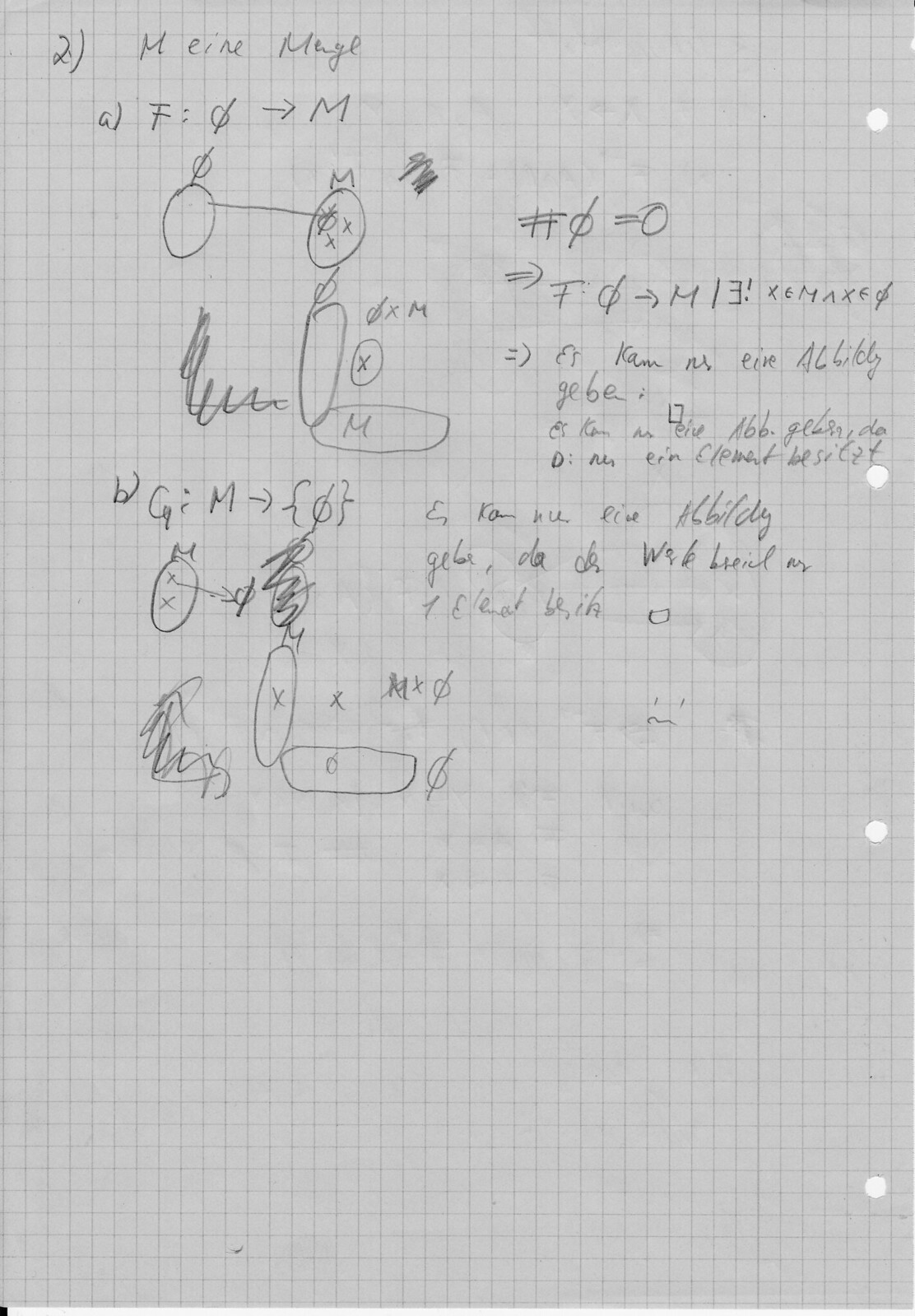The image depicts a meticulously detailed sheet of graph paper, characterized by an off-white or slightly grayish hue and intersecting gray lines that form a grid of hundreds of tiny squares. Notably, the paper has four evenly spaced holes punched along its right side, suggesting it has been flipped over for use.

At the top left corner, the sheet begins with the notation "2)" followed by text in what appears to be a foreign language: "MEINE MAGE." Further down, an equation or notation starts with "A)" followed by "F:" and the null symbol (Ø) leading to an "M."

The center of the page features a series of interconnected sketches, including circles and ovals that are arranged both horizontally and vertically. Some of these shapes contain marked Xs within them, adding to the cryptic nature of the document. Along the right side of the paper, there is additional text in the same foreign language, including fragments like "ES KAM NR EISE," among others.

Overall, the page is filled with a variety of mathematical calculations, sketches, and annotations, combining to create a dense and complex visual representation of analytical work.